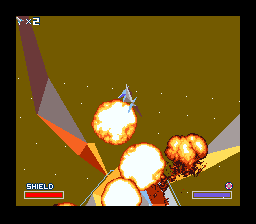The image is a screenshot from a retro game, possibly from the late 80s or early 90s, characterized by its dated graphics. The scene is chaotic with five distinct explosions, creating a dynamic and intense atmosphere. Above one of the explosions, a dragon-like creature with vibrant, multi-colored wings in shades of orange, purple, yellow, and gray appears to be flailing, as if it has been forcefully ejected. The background is a muddy brown, invoking a gritty, otherworldly environment. The game’s interface displays a "shield" bar in red and another bar with a different symbol in blue, likely indicating the player's health or energy. In the top-left corner, a character icon is shown with "x2," suggesting extra lives or a multiplier.